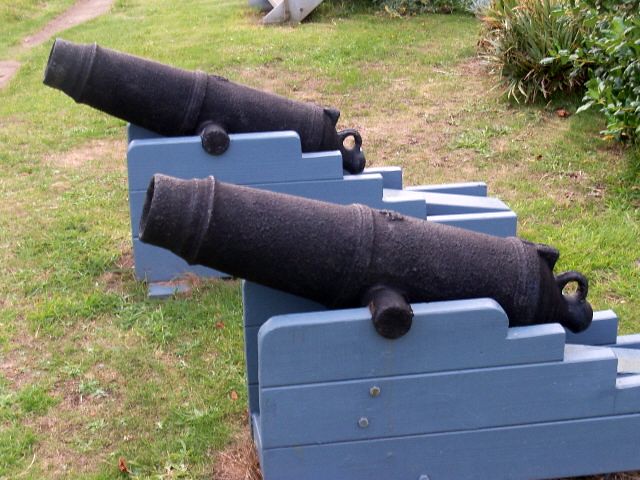The image captures a close-up view of two old-fashioned, black cast iron cannons, which are short and slightly bumpy in texture. The cannons are positioned outdoors on a patchy green field, indicating less well-maintained grass, possibly during the spring or summer months. They rest on light blue platforms, made either of wood or a durable plastic-like material, specifically designed for them. The cannons are identical and are stacked close together, pointing towards the top left of the image with their barrels slightly tilted upwards. In the background, one can observe bushes with hints of yellow, a sliver of a dirt path in the top left corner, and part of a wooden staircase, adding to the historical ambiance of the scene.